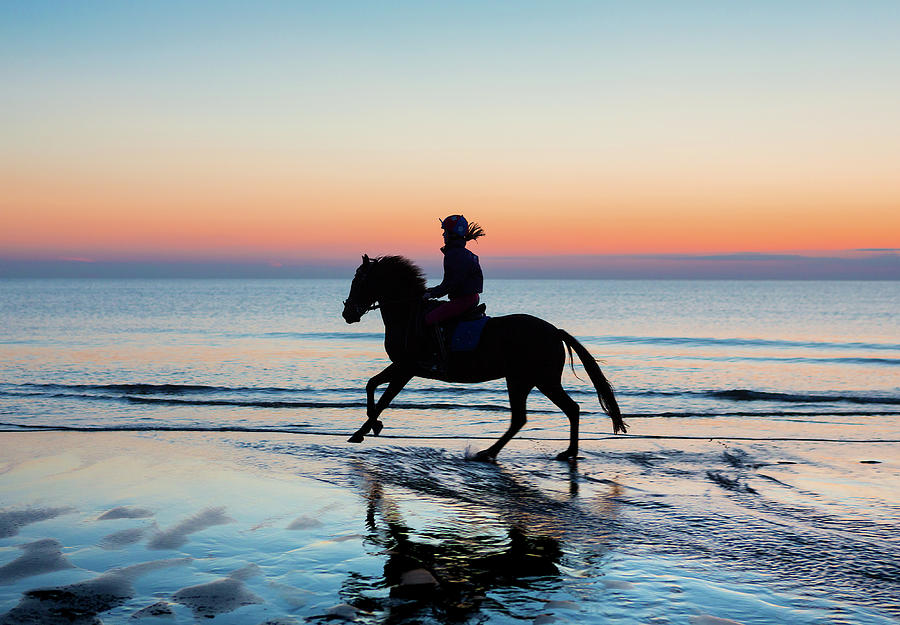The image captures a serene scene of a person riding a horse on a beach during twilight. The horse, positioned centrally in the photograph, is trotting on the wet part of the beach, where small, calm waves are reaching the sand. Both the horse and rider are silhouetted in black, obscuring details but highlighting the rider's long hair and blue helmet. The beach's dark tone contrasts with the gentle blue of the ocean, which appears vast and extends into the horizon. The twilight sky is a blend of deep blue at the top transitioning through light orange to a darker, golden hue closer to the horizon, with dark gray clouds scattered at the bottom, indicating the setting sun behind them. The overall atmosphere is tranquil, capturing the peaceful interaction between the rider, horse, and the natural coastal landscape.